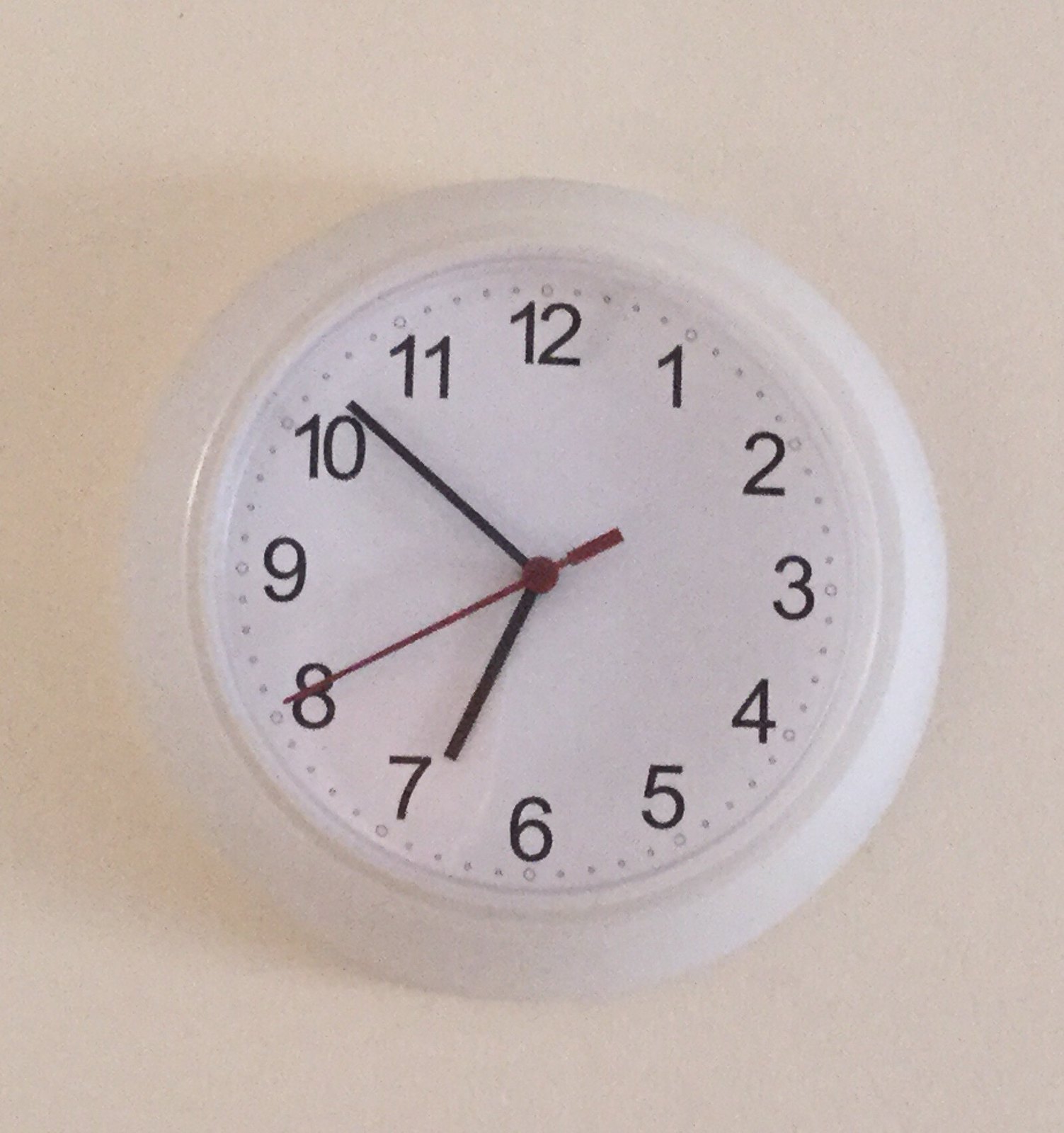The clock features a light-bodied, white face adorned with numerals 1 through 12 arranged in a traditional clockwise sequence. Encircling the numeral track are two sets of dots, with the larger circle dots encompassing the entirety of the clock face. The red second hand, designed with a distinctive large rectangular tip, points precisely at the 8. The hour hand is positioned at the 7, while the minute hand lies between the 10 and 11 markers. At the center of the clock, a dot secures the hands, creating a focal point. A shadow is cast upon the clock face, indicating an external light source. Additionally, the subtle reflection hints that the clock might be encased in plastic or glass.